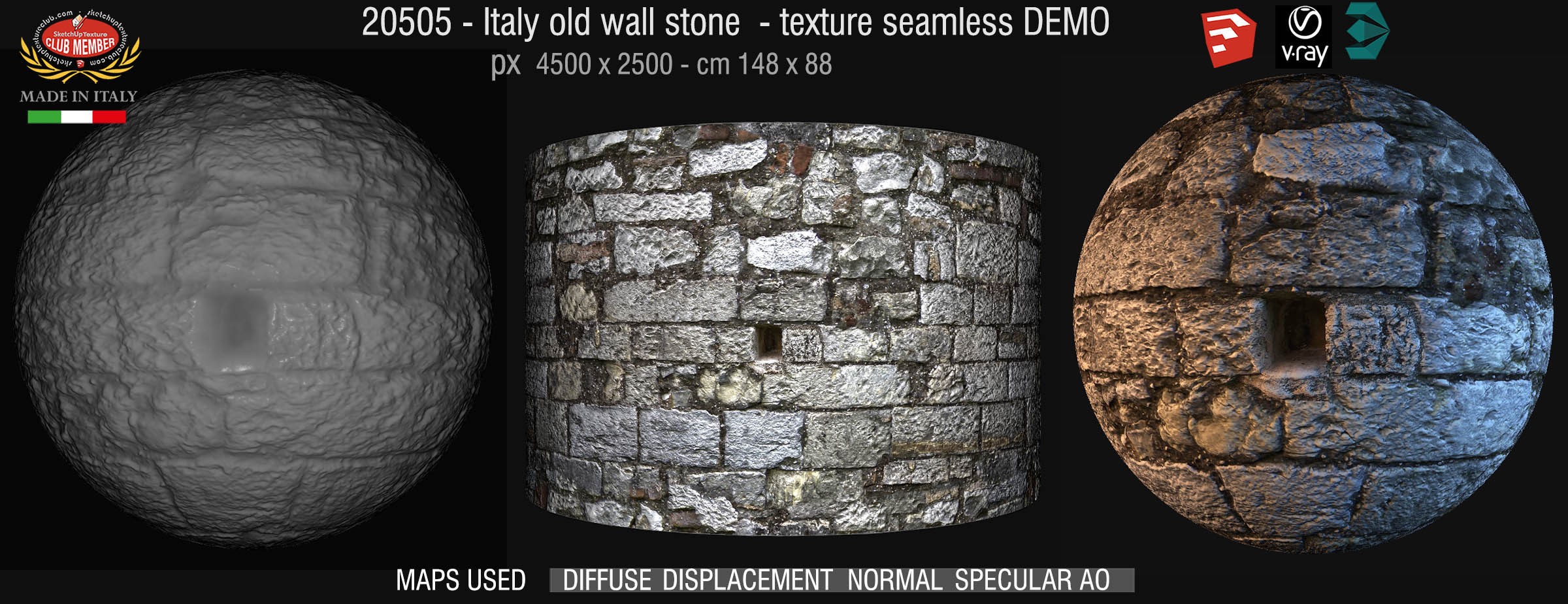This computer-generated image features a black background with a prominent white text at the top center reading "20505 - Italy old wall stone - texture seamless demo." Below this text, another notation specifies "PX 4500 x 2500 - centimeters 148 by 88." In the top-left corner, an Italian flag is displayed alongside a logo with the text "Made in Italy." The image showcases three distinct structures composed of brick textures and varied shapes: on the left is a spherical object with a brick pattern, in the center is a cylindrical object featuring gray and green bricks, and on the right is another spherical object made up of larger, rectangular gray and green bricks. At the bottom center of the image, the text reads "maps used: diffuse, displacement, normal, specular, AO."